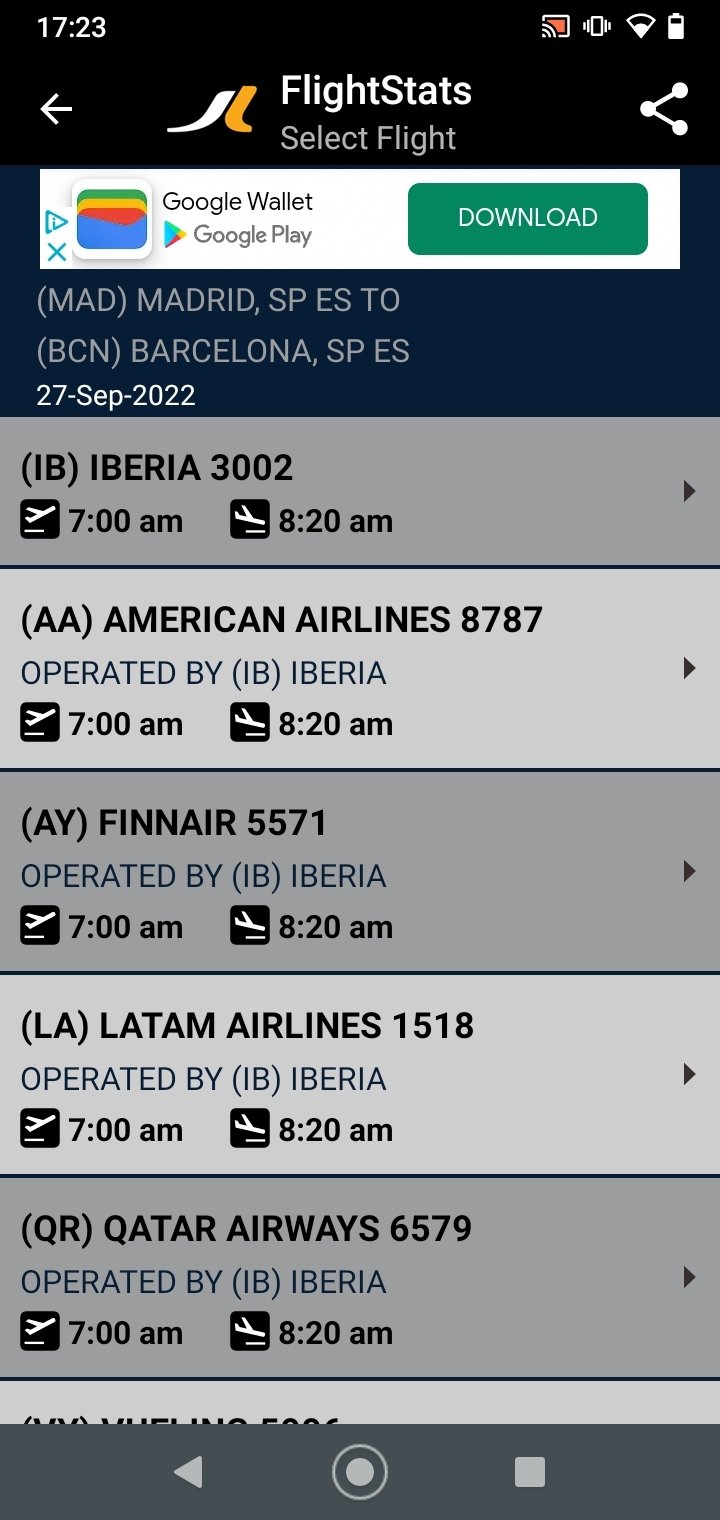The screenshot captures a travel app displaying details for flights. In the top left corner, the current time is shown as 17:23, while the top right corner indicates the Wi-Fi and battery status. The main header of the app reads "Flight Stats" followed by "Select Flight." Directly below, there's an advertisement for Google Wallet. 

The flight details section lists a journey from Madrid (MAD) to Barcelona (BCN) on September 27, 2022. Beneath this, several flight options are presented with identical departure and arrival times of 7:00 AM to 8:20 AM. The options are:

1. Iberia (IB) flight 3002
2. American Airlines (AA) flight 8787, operated by Iberia
3. Finnair (AY) flight 5571, operated by Iberia
4. LATAM Airlines (LA) flight 1518, operated by Iberia
5. Qatar Airways (QR) flight 6579, operated by Iberia

Each option follows a consistent format, indicating the primary airline and any operational partnerships.